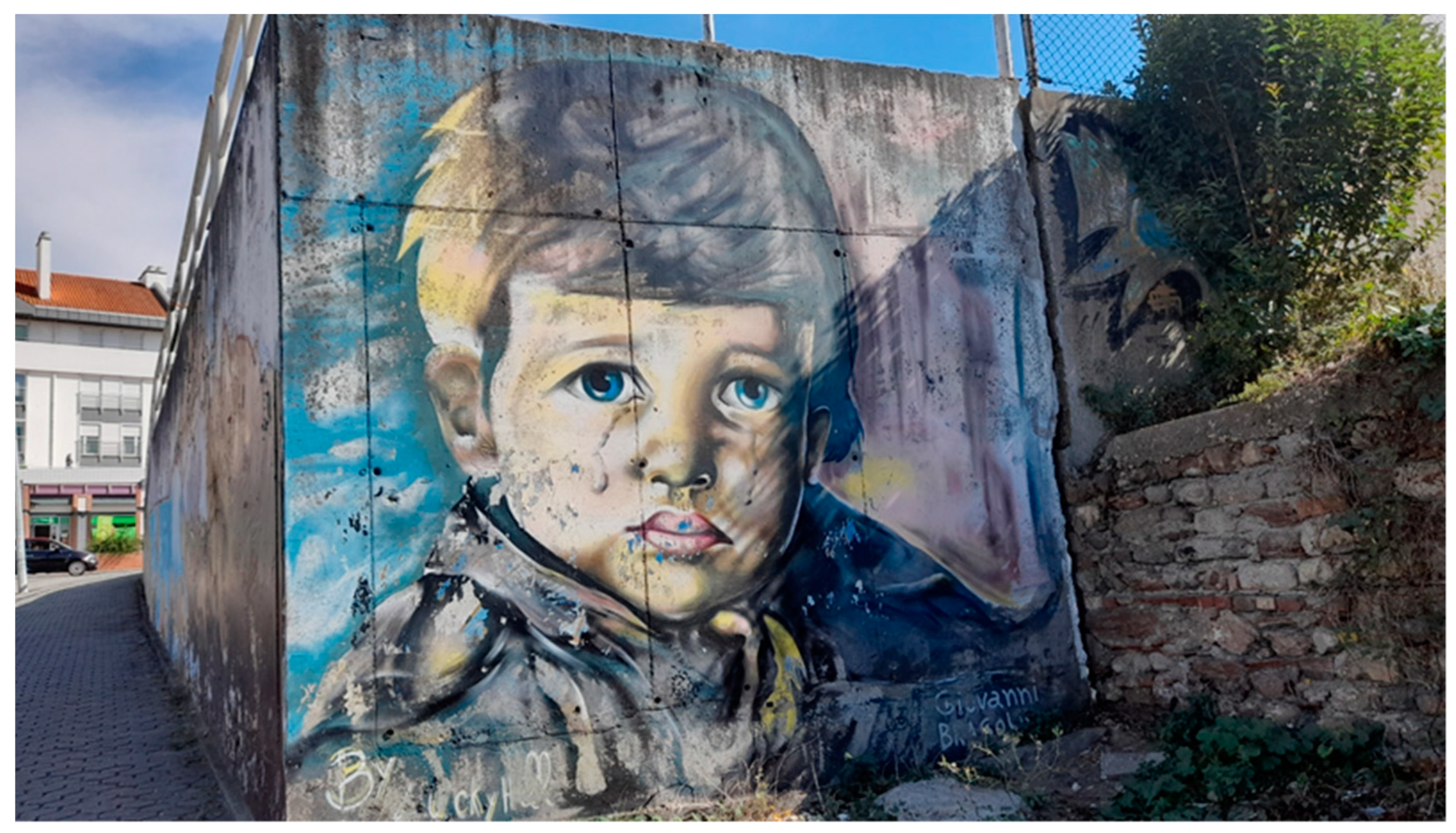This image features a large, outdoor mural centered on a concrete wall, approximately 8 to 10 feet square. The mural depicts a young Caucasian boy with intensely bright blue eyes, which appear to be staring out at the world with a look of deep concern or fear. Tears stream down his face, and his reddish lips contrast sharply with his blond, neatly combed hair. The boy is wearing a grey winter coat and is framed by a blue aura emanating behind him, against the blue background of the mural.

On the right side of the image, there's an older stone wall with some vegetation and a tree, while the left side shows a street, possibly in front of a storefront and a house. Beyond that, a horizon is visible with a larger apartment-like building and a clear blue sky. The bottom of the mural bears the name of the artist, which appears to read "Lucky Hall."